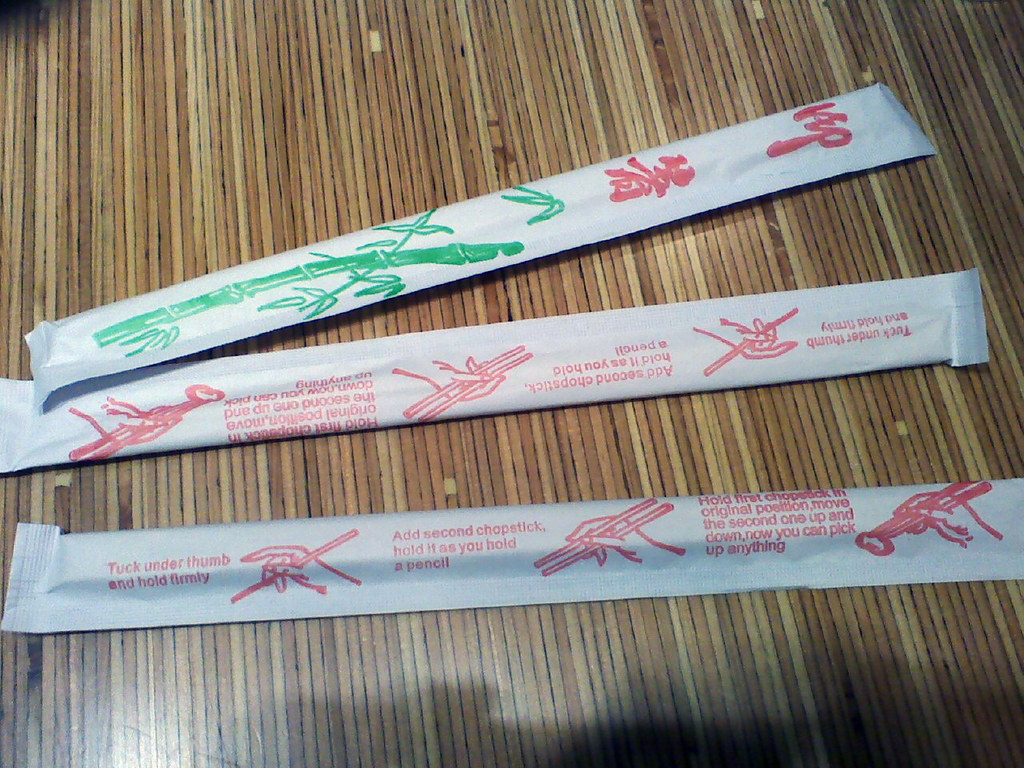A detailed photograph showcases three individually wrapped packages of chopsticks from a Chinese restaurant, arranged horizontally on a rustic wooden table with thin, straw-like wooden strips. Each chopstick wrapper is white, adorned with red ink. The top wrapper, oriented at an angle, features two Chinese characters and a simple graphic of a green bamboo shoot. The two lower wrappers are identical and positioned with their instructional text visible. These wrappers instruct on proper chopstick use, with diagrams illustrating each step: "Tuck under thumb and hold firmly," "Add second stick, hold it as you would a pencil," and "Hold the first chopstick in the original position, move the second one up and down." The final diagram shows an item being picked up by the chopsticks. The wrappers' text and images are all in red ink, contrasting against the white paper. The second wrapper is upside down, mirroring the bottom one.